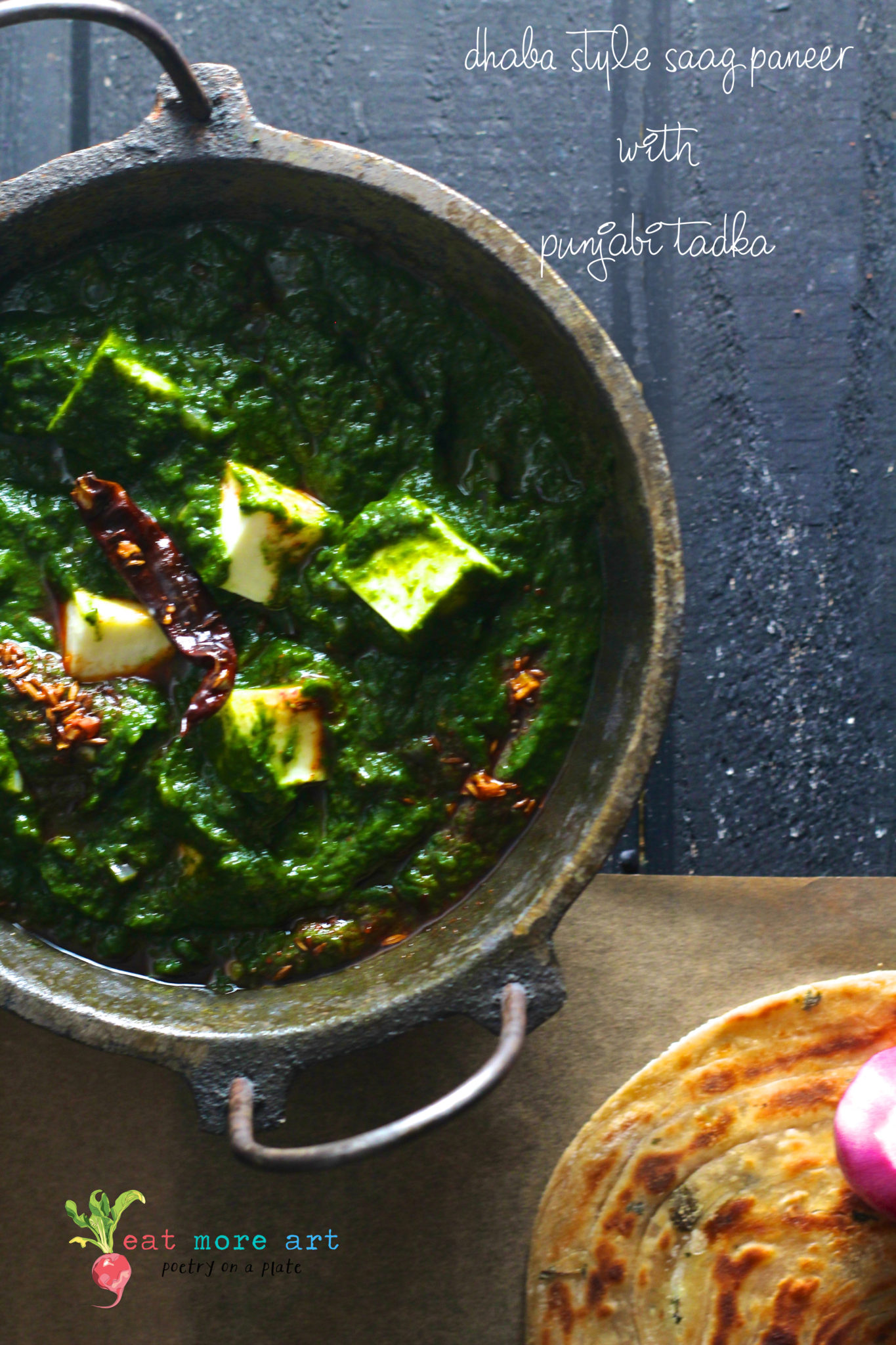The image is a vibrant advertisement featuring a top-down view of a rustic, heavy metallic silver pot with arched handles in a rusted hue, positioned slightly left of center. Inside the pot, there's a vividly green, mushy dish topped with white cubes and a singular orange chili piece. The backdrop on the right side is a dark blue with scattered white speckles, creating a rough-edged appearance. Handwritten in white text at the top of the image are the words “Dhaba Style Saag Paneer with Punjabi Tadka.” At the bottom left, there is an illustration of a radish with green leaves and a red root, accompanied by the phrase “Eat More Art,” where “Eat” is in red, “More” in teal, and “Art” in blue. In the bottom right corner, a round piece of yellow flatbread with brown spots is visible, adding a final touch to the culinary display.